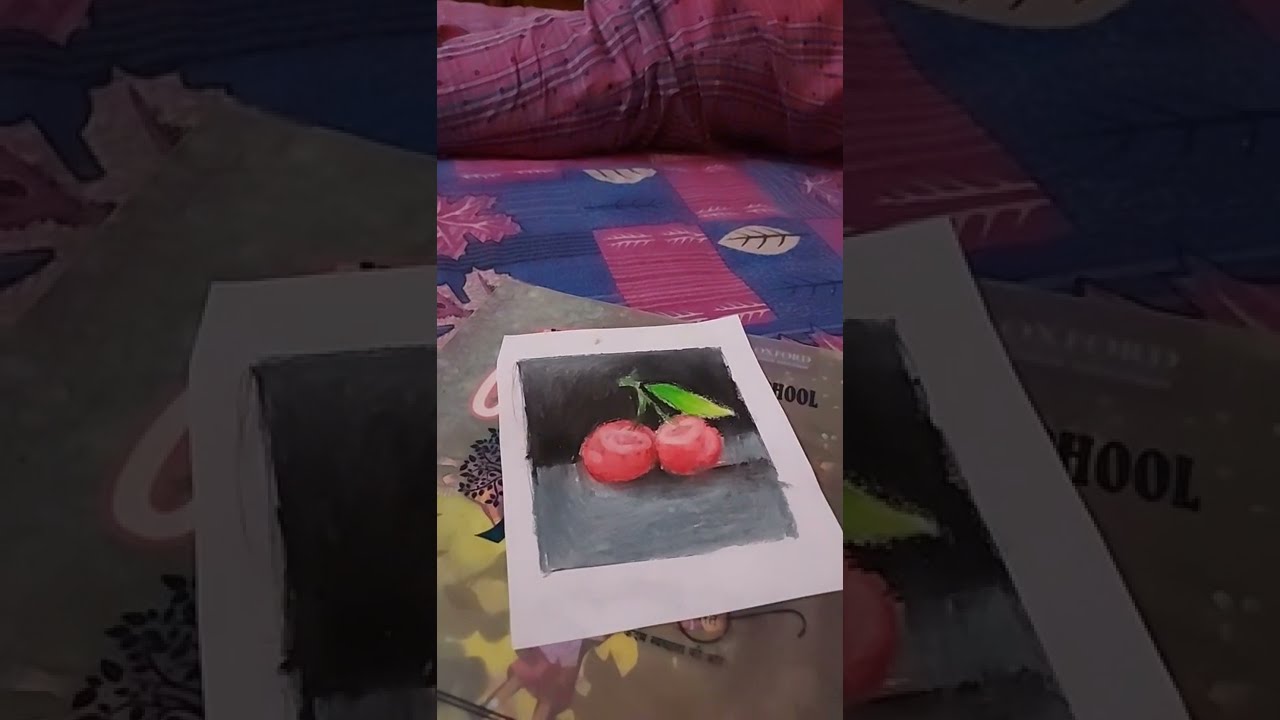In the center of the image, we see a detailed painting of two red cherries connected by green stems with a single green leaf. The cherries are positioned against a black background and appear to be resting on a gray table. This vibrant painting is on a white piece of paper, which is sitting atop a larger, more complex background. Surrounding the piece of paper is another painting or print, characterized by gray and yellow hues. Beneath and around this setup is a visually rich bedspread with a pattern of blue and red squares and white and red leaves. This bedspread seems folded over, revealing another layer with pink and blue squares and tan leaves, and parts of this fabric extend into the background of the image. Additionally, in the background, there's a black and red striped blanket. The left and right edges of the main painting feature blown-up, darkened versions of the cherry image, reminiscent of the style often seen in TikTok reels. The intricate layering and varied textures, from the cherries' painting to the detailed fabric patterns, create a visually engaging composition.